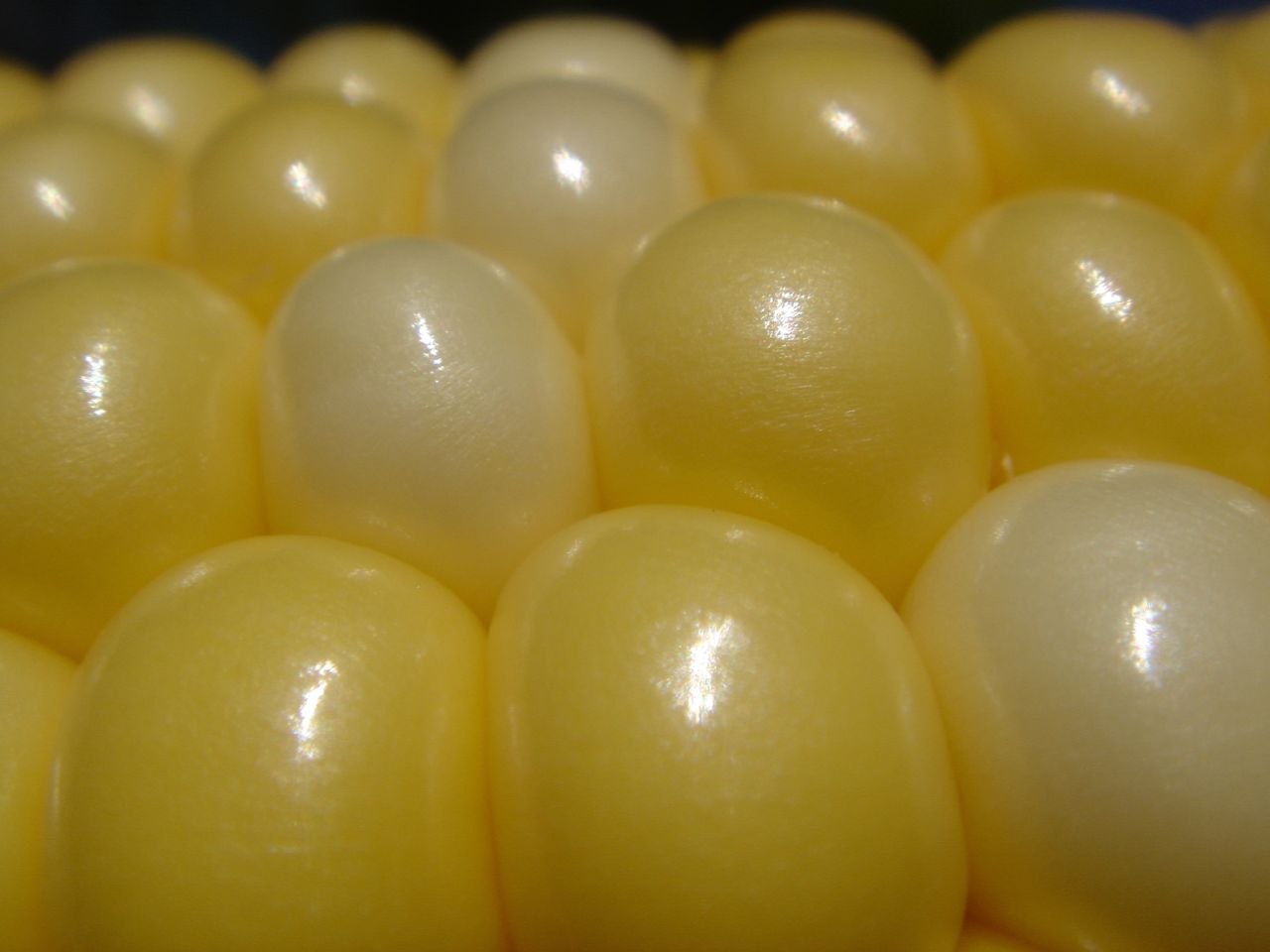The image is a large, square, close-up color photograph featuring approximately 15 smooth, rounded objects resembling balloons or candies, primarily yellow with a few being white or ivory. The objects are packed closely together, creating an overlapping pattern with noticeable light reflections where the light source hits them. In the bottom row, three objects are visible: two yellow on the sides and one white in the center. The row above has four objects: a yellow, a white, and two yellows. The next row, which starts to blur into the background, contains five objects: two yellows, a white in the middle, and two more yellows. At the very top, there is a thin strip of pure black, indicating the background. The objects appear soft, potentially squeezable, and perhaps made of rubber, despite their visual similarity to balloons or candies.